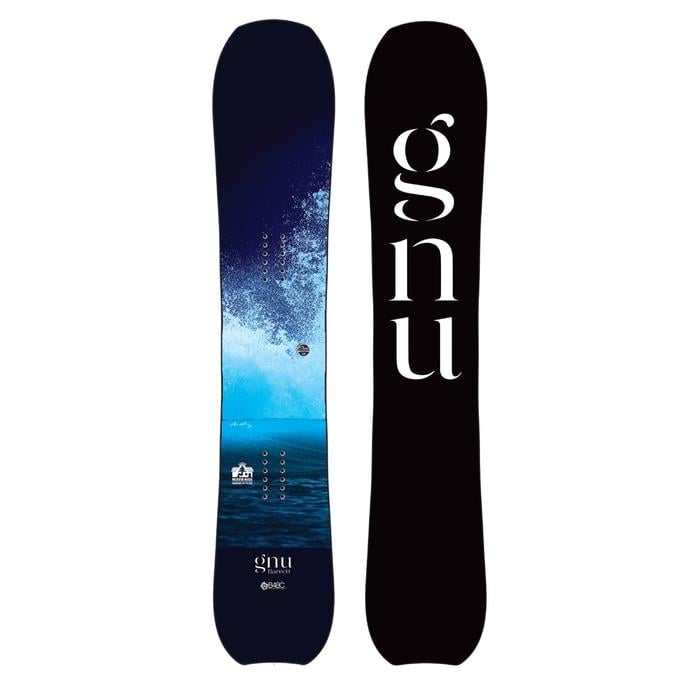The image features a pair of water skis centered against a plain white background. The left ski showcases an oceanic theme with an image of crashing waves, a sky, and bubbles, while the word "GNU" appears in small print near its bottom. The right ski is predominantly black and also bears the word "GNU" in white letters. Both skis include attachment points that suggest foot bindings, reinforcing their function as water sports equipment. The skis are displayed flat, side by side, and their sleek, thin design is indicative of high-performance water skis. The combination of colors—white, black, dark blue, light blue, and gray—adds to the dynamic and sporty aesthetic, making this image suitable for a sporting goods advertisement.